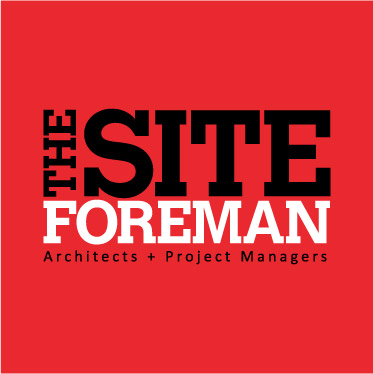The image features a square-shaped banner with a muted red background. Prominently displayed in the center, large black text spells out "the site," with "the" oriented vertically and "site" horizontally beside it. Directly beneath, in bold white capital letters, is the word "FOREMAN." Below this, in much smaller black print, are the words "Architects + Project Managers," with each word beginning with a capital letter. The design uses a mix of large and highly readable fonts to emphasize different elements, likely serving as an advertisement for a construction or architectural project seeking a foreman.